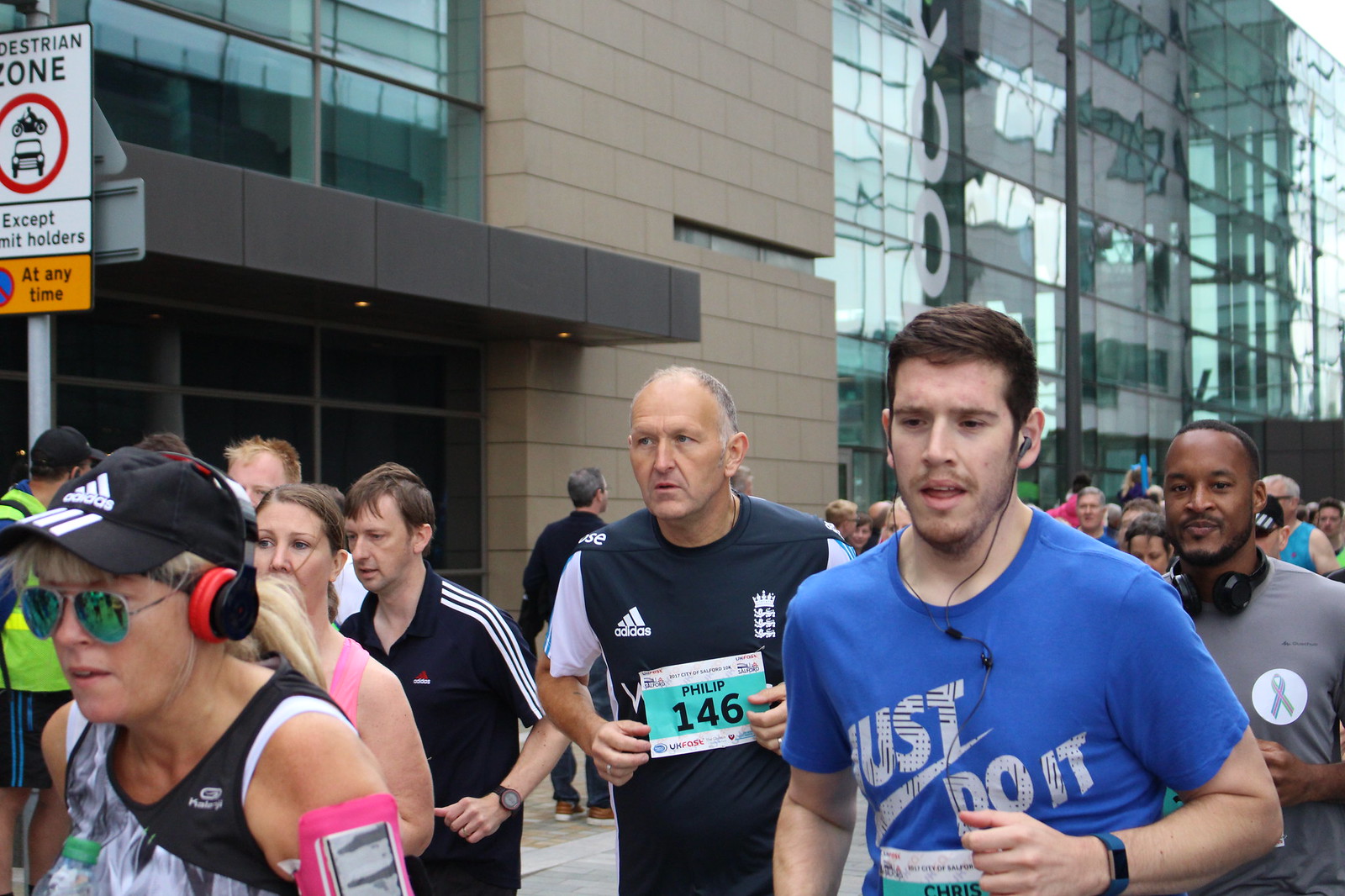The image captures a dynamic moment from a marathon taking place on a city street. A diverse group of runners of varying ages and genders is prominently featured, all heading towards the left. The central focus is on a young white male wearing a blue Nike "Just Do It" t-shirt, who is running alongside an older male, approximately 60 years old, dressed in a black Adidas shirt with the name "Philip" and number 146 displayed on his front. Next to them is another runner, a black male in a grey shirt, sporting headphones around his neck. The race appears non-professional, possibly a charity or corporate event, given the casual demeanor of the participants.

In the background, a tall building with distinctive blue-green glass towering over the streets is visible, reminiscent of a mall or a commercial complex. To the upper left, a street sign marking a pedestrian zone with an exception for permit holders is noticeable. There is a mix of onlookers in the vicinity, some walking in the opposite direction, disengaged from the race. The surrounding environment includes another beige and black building with extensive glass frontage, adding to the urban vibe of the scene.